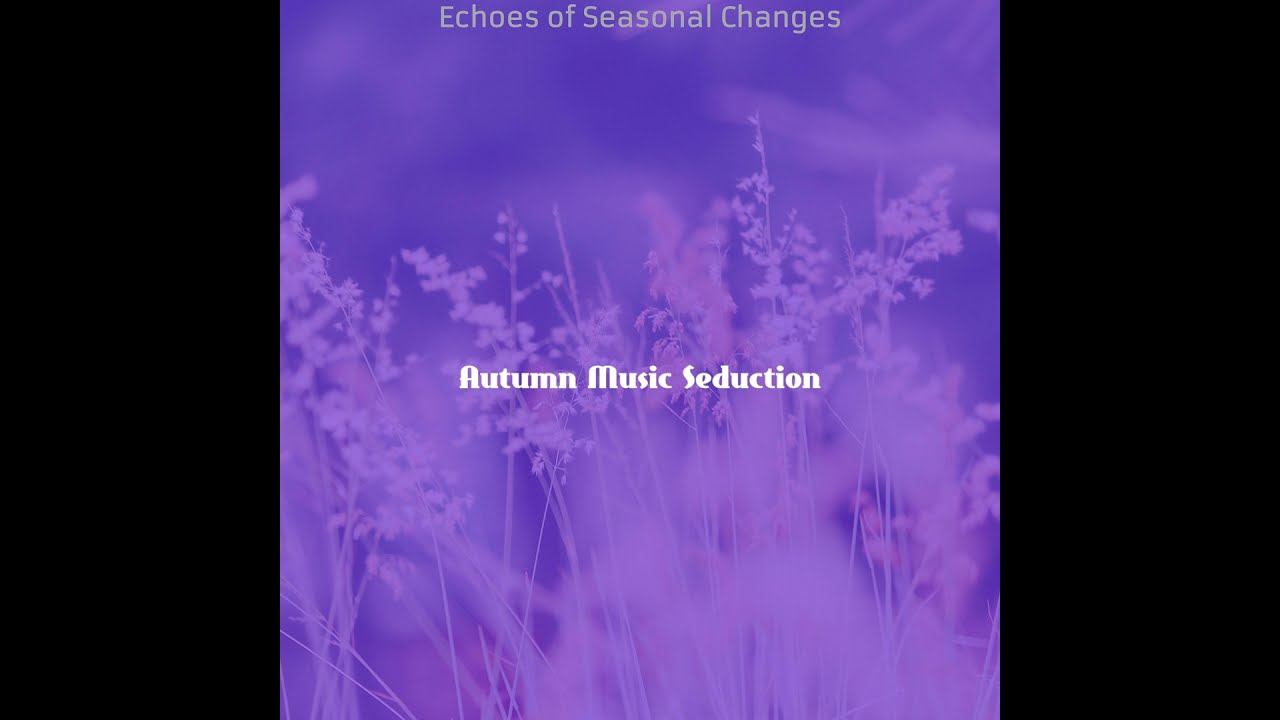The image resembles a CD cover, framed by thick black borders on the left and right sides. The center is dominated by a pale purple background, featuring subtle hues of light and dark blue. At the very top, in gray letters, it reads, "Echoes of Seasonal Changes." Centrally placed in the composition, "Autumn Music Seduction" is prominently displayed in bright white text. The background showcases a photograph of a field with various floral plants, characterized by stalks adorned with clusters of small flowers. The overall image is tinted with a purplish hue, obscuring the true colors of the flowers and plants, which might include lighter shades like yellows, pinks, and purples.